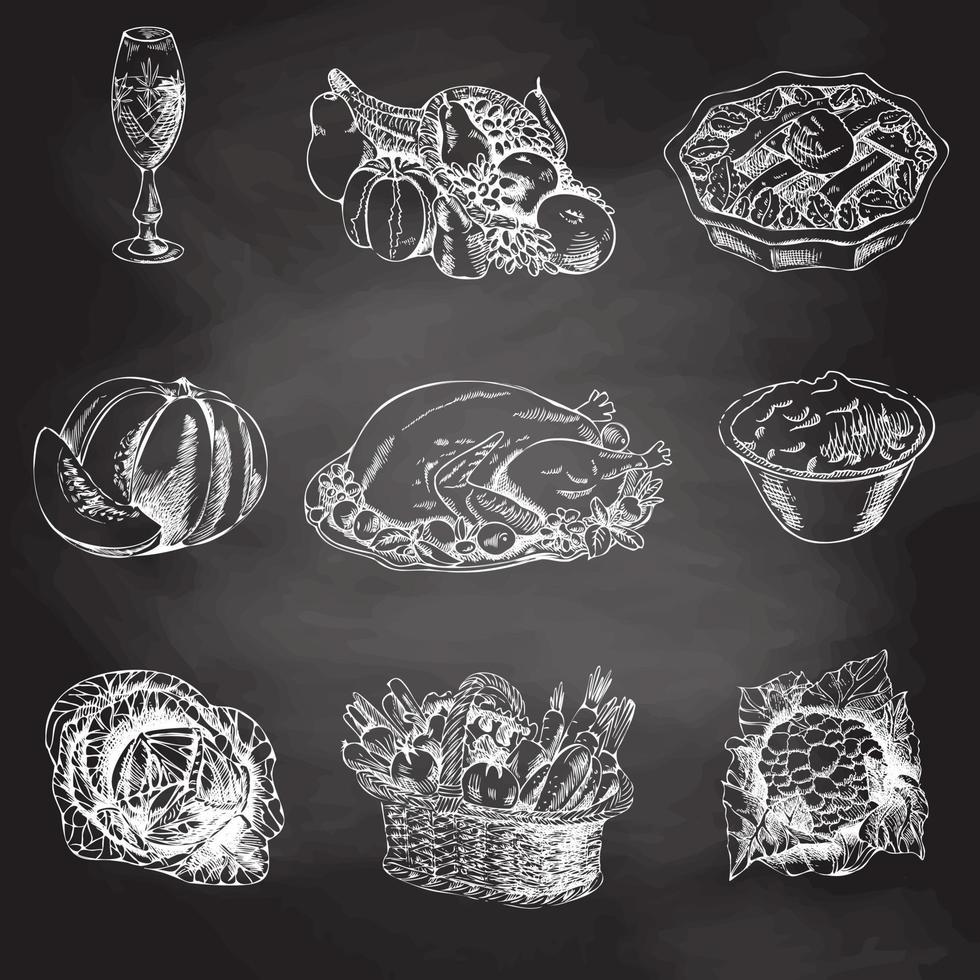The illustration features a black or dark gray background adorned with intricate white pencil drawings, each carrying a faint glow. Centered on a subtly lighter gray patch, these images appear to portray elements of a festive feast, possibly Thanksgiving. At the top left, there is a wine glass detailed with elegant etchings, similar to a champagne flute. Beside it, in the upper middle, is a cornucopia spilling over with pumpkins, squash, grapes, and other fruits. On the top right, an apple pie is depicted with a lattice crust. In the middle row on the left, a pumpkin with a wedge cut out sits next to its missing piece, while the centerpiece of this row is a cooked turkey presented on a platter, surrounded by an assortment of fruits and vegetables. To the turkey's right, a bowl possibly containing mashed potatoes or jello is positioned. The bottom row features, from left to right, bundled lettuce or cabbage, a wicker basket overflowing with vegetables such as carrots and radishes in the middle, and an illustration of a cauliflower or another leafy vegetable on the far right. The entire scene is framed elegantly, evoking a sense of a lavish Thanksgiving spread.